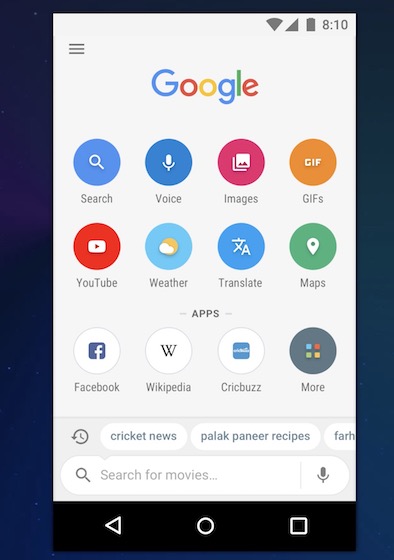This image displays a smartphone home screen prominently featuring the Google logo centered at the top. In the top right corner, the time is shown alongside a battery indicator and a Wi-Fi signal icon. 

The screen is populated with several interactive options, each represented by colorful circles with specific icons and labels:

1. A blue circle with a white magnifying glass labeled "Search."
2. A darker blue circle with a white microphone labeled "Voice."
3. A bright purple circle labeled "Images."
4. An orange circle labeled "GIFs."
5. A red circle featuring a white play button labeled "YouTube."
6. A light blue circle with a sun and cloud emblem labeled "Weather."
7. A dual-character icon with an 'X' and an 'A' labeled "Translate."
8. A green circle labeled "Maps."

Below these options, the screen transitions into a section with a variety of app icons, including Facebook, Wikipedia, and CirqBuzz, with an additional "More" button available for accessing more apps.

A white search field is prominently positioned for inputting queries, accompanied by a microphone icon for voice searches. The search history is displayed within the field, with recent entries such as "cricket news" and "paneer recipes" visible.

This comprehensive assortment of features and tools showcases the versatile functionality available directly from the smartphone’s home screen.